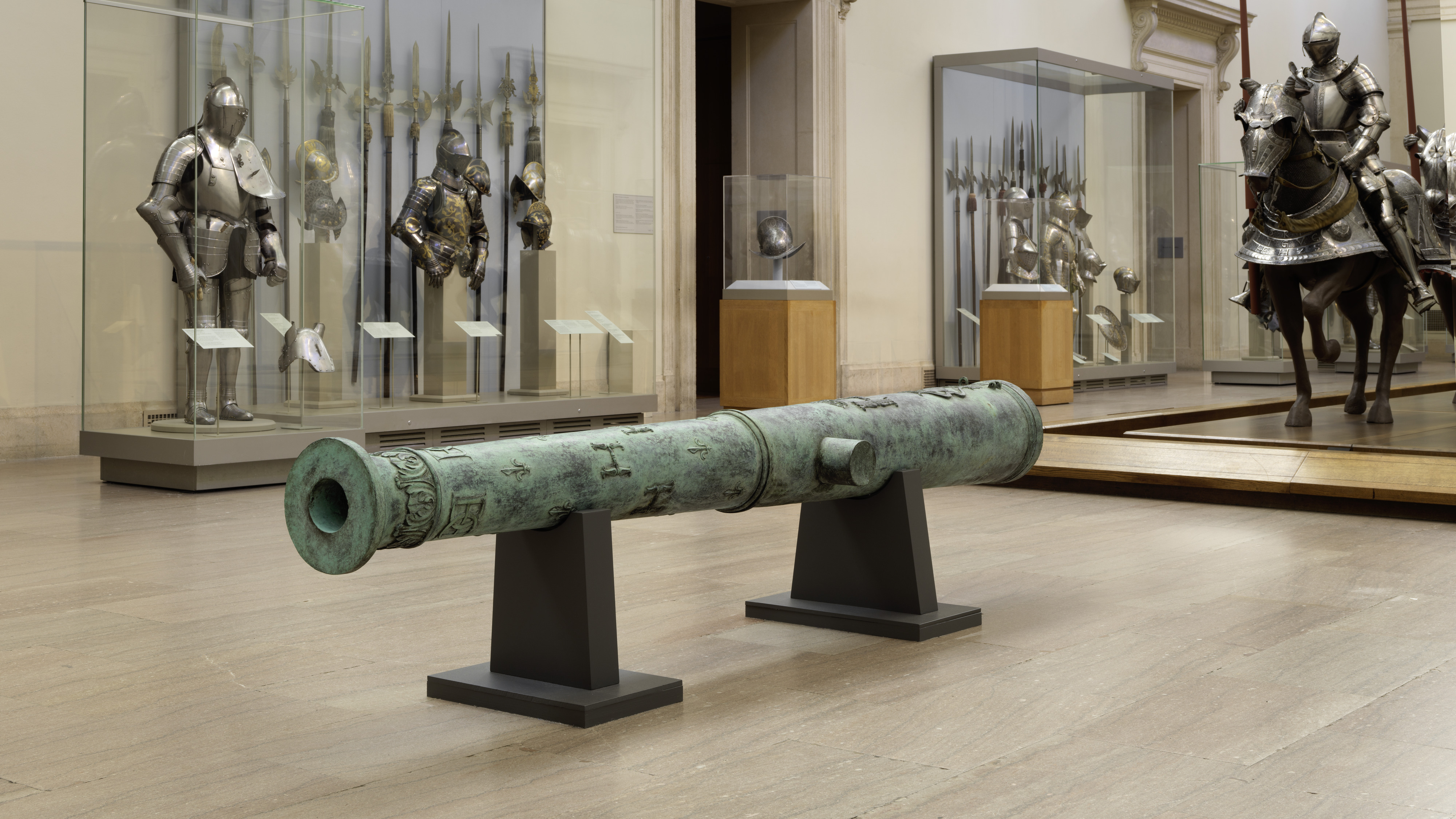The image depicts the interior of a well-lit history museum or art gallery, showcasing a detailed collection of medieval and war artifacts. The room is meticulously arranged with brightly colored items housed in glass display cabinets and mounted on sturdy stands. The foreground features a prominent battering ram, likely used to breach castle doors, sitting on thin black pillars fixed into the smooth, clean floor.

Dominating the background is a lifelike display of a horse clad in full armor, with one leg raised to simulate movement. An armored figure sits astride the horse, holding a spear in the right hand. Surrounding this central exhibit are various other items: armors, cannons, helmets, shields, and medieval weapons like spears, all elegantly placed to illustrate their historical significance.

The left side of the image features more armor and weaponry, with items positioned both on the walls and in individual glass cases. The colors in the room range from beige and brown to gray, silver, bronze, black, and green, with the lighting enhancing the visibility and details of each artifact.

This comprehensive arrangement suggests a focus on medieval warfare, knight armor, and historical battles, offering visitors a rich visual narrative of past conflicts and combat technologies.